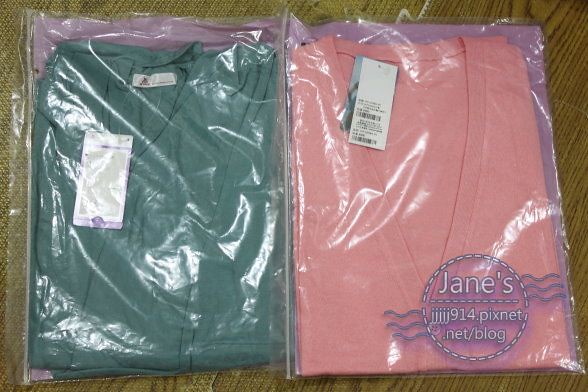In this image, two packs of shirts are displayed on a medium-brown wooden table with visible wood grain. Both shirts are tightly folded and encased in individual clear plastic packaging, which has a light purple background. On the left side, there is a green shirt, possibly a t-shirt with a thin material, and a dark purple shirt folded behind it. This shirt has both a visible tag at the back of the neck and a rectangular white price tag hanging at the front. The right side features a salmon pink shirt with a deep V-neck, also made of a thin fabric, with a purple shirt similarly folded behind it. This shirt has a matching white price tag on the front. On the bottom right corner of the pink shirt's package, there is a circular logo outlined in purple with the text "Janes, jjjjj914.picsnet.net/blog" in white, and is accompanied by wavy purple designs on either side.